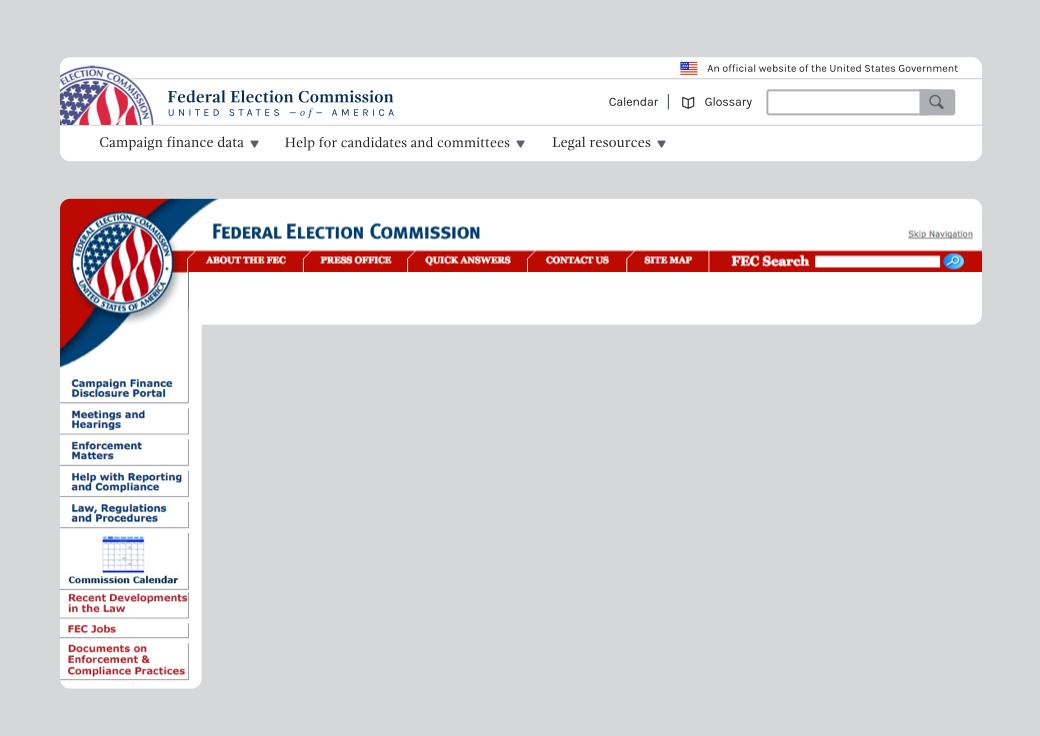This is a detailed visual description of the homepage of the Federal Election Commission (FEC) website of the United States of America.

---

The FEC website prominently features a patriotic theme with a color scheme of red, white, and blue. At the top right-hand side of the page, there is a statement, "An official website of the United States government," accompanied by an image of the American flag. On the left-hand side, the Federal Election Commission logo is displayed, featuring an emblem that incorporates the American flag. 

Beneath the header, three main navigational options are presented in black: "Campaign Finance Data," "Help for Candidates and Committees," and "Legal Resources." Each of these options includes a drop-down arrow for additional information or options. Nearby, the website offers a calendar, a glossary, and a search bar for specific inquiries.

Highlighted in blue letters below, the text "Federal Election Commission" appears, along with a "Skip Navigation" option for accessibility. The FEC seal, with the text "Federal Election Commission United States of America" encircling the American flag, can be seen, accentuated by red and blue stripes.

Further navigation options are presented below. Red-bordered buttons with white lettering provide links to "About the FEC," "Press Office," "Quick Answers," "Contact Us," "Sitemap," and "FEC Search." 

On the left-hand side, under the FEC logo, additional options are displayed. Written in blue on a white background, these include "Campaign Finance," "Disclosure Portal," "Meetings and Hearings," "Enforcement Matters," "Help with Reporting and Compliance," and "Law Regulations and Procedures." 

At the bottom of the page, recent developments and resources are outlined in red text on a white background. These include "Recent Developments in the Law," "FEC Jobs," and "Documents on Enforcement and Compliance Practices."

---

This detailed description captures the layout, visual elements, and navigational structure of the Federal Election Commission’s website homepage.